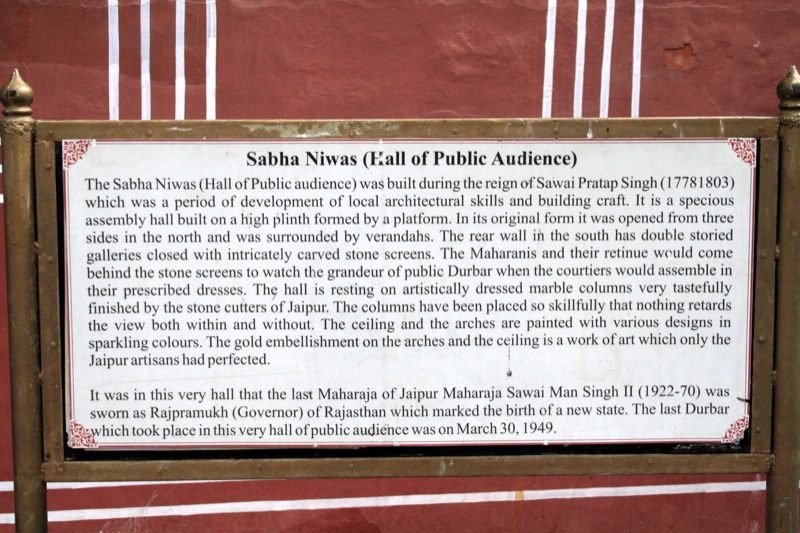The photograph showcases a close-up view of a commemorative signboard set against a dark mulberry or burgundy wall with white stripes. The signboard, framed in a rectangular brown painted frame with two round poles on either side, is made of metal and wider than it is tall. The surface of the sign features black text on a white background, with some reddish embroidery decor at the corners. It reads prominently in bold letters, "Sabha Niwas, Hall of Public Audience."

The sign details the historical significance of Sabha Niwas, an expansive assembly hall built during the reign of Sawai Pratap Singh between 1778 and 1803. This period marked the development of local architectural skills and building craftsmanship. The hall, originally open on three sides to the north and surrounded by verandahs, stands on a high plinth platform. The rear southern wall features double-storied galleries enclosed with intricately carved stone screens.

Further descriptions highlight that the hall's ceiling and arches are adorned with vivid designs and golden embellishments, showcasing the artistic prowess of Jaipur's stone cutters and artisans. The marble columns, skillfully placed, allow an unobstructed view within and without.

The sign also commemorates significant historical moments, such as the swearing-in of the last Maharaja of Jaipur, Maharaja Sawai Man Singh II (1922-1970), as the Rajpramukh (Governor) of Rajasthan, marking the birth of a new state. The last Durbar in this hall took place on March 30th, 1949.